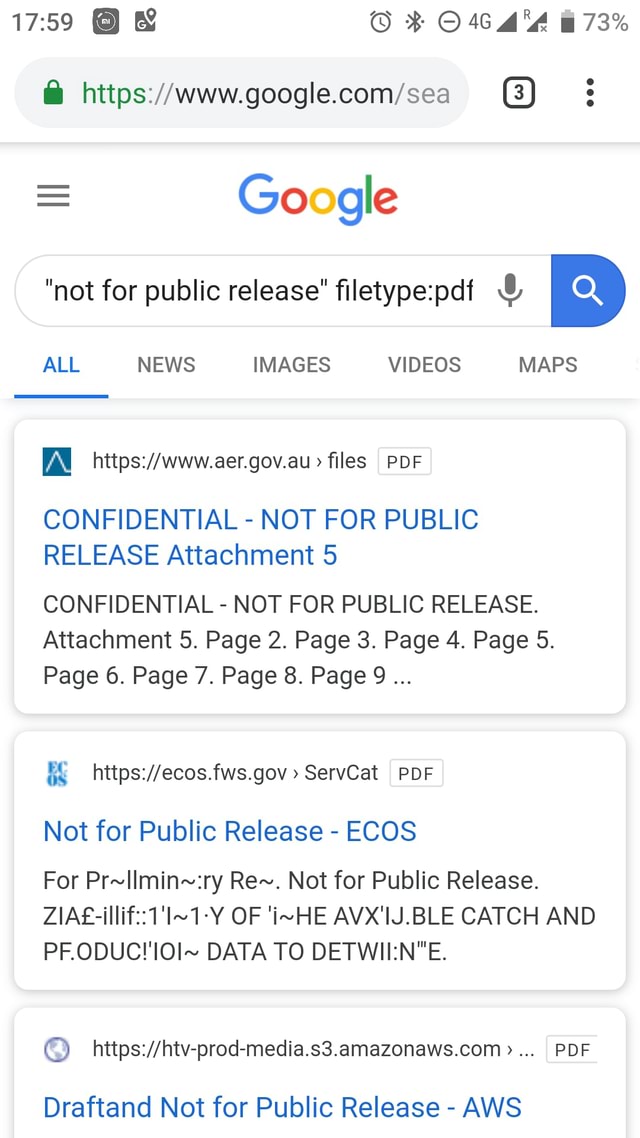The image displays the Google web search page in great detail. At the top of the screen, the military time reads 17:59. Adjacent to the time, there's an icon resembling a square with a circle inside it, accompanied by some type of text. Next to this icon is what appears to be a Google Maps icon. Centrally located near the top-middle area, there are various icons including a clock, Bluetooth, a circle with a minus sign, the 4G network indicator, and multiple signal strength bars, both showing full strength. One of the signal areas includes an "R" at the top and an "X" at the bottom. The battery life indicator shows 73% remaining.

The address bar begins with "HTTPS," accompanied by a green lock icon, indicating a secure connection. Below the address bar, there is a three-line menu icon (often referred to as the hamburger menu). Prominently featured in the middle of the page is the Google logo, with its familiar blue, red, yellow, and green colors. Within the address bar, the text reads "not for public release, file type: PDF."

Lower on the page, the navigation options "All," "News," "Images," "Videos," and "Maps" are visible, with "All" highlighted in blue. Below this menu, the search results start with a heading marked "Confidential, not for public release," followed by "Attachment 5: Confidential, not for public release." Additional text entries also state "not for public release," and the phrase "drafted not for public release" is partially visible, being cut off at the end.